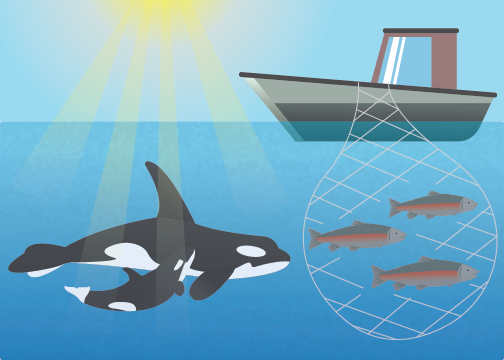This vibrant illustration, presented in landscape orientation, vividly depicts an underwater scene featuring a mother killer whale and her baby. The black and white mammals are seen swimming from left to right, positioned at the bottom of the image. Surrounding them, the water is predominantly blue, revealing various hues where sunlight penetrates. The sun is located in the upper left corner, emitting radiant beams that extend downwards, casting illuminating streaks through the water and subtly altering the appearance of the whales wherever the light touches.

To the upper right, a simple, two-layered fishing boat floats on the surface. The boat, characterized by a darker gray hue at its submerged portion, transitions to a lighter gray and is topped with a distinct red and blue area, including a noticeable blue windshield. Draped over the boat's side is a white mesh fishing net, clearly discernible by its crisscross pattern.

Caught in this net are three small fish, each gray with distinctive red stripes, oriented toward the right side of the image. The dynamic interaction suggests a sense of pursuit and curiosity, possibly frustration, as the mother whale appears focused on the entrapped fish, unable to reach them due to the net. This scene, rich in detail and energy, is vividly brought to life through the illustrative and lightly cartoonish style, merging elements of both realism and artistic interpretation.